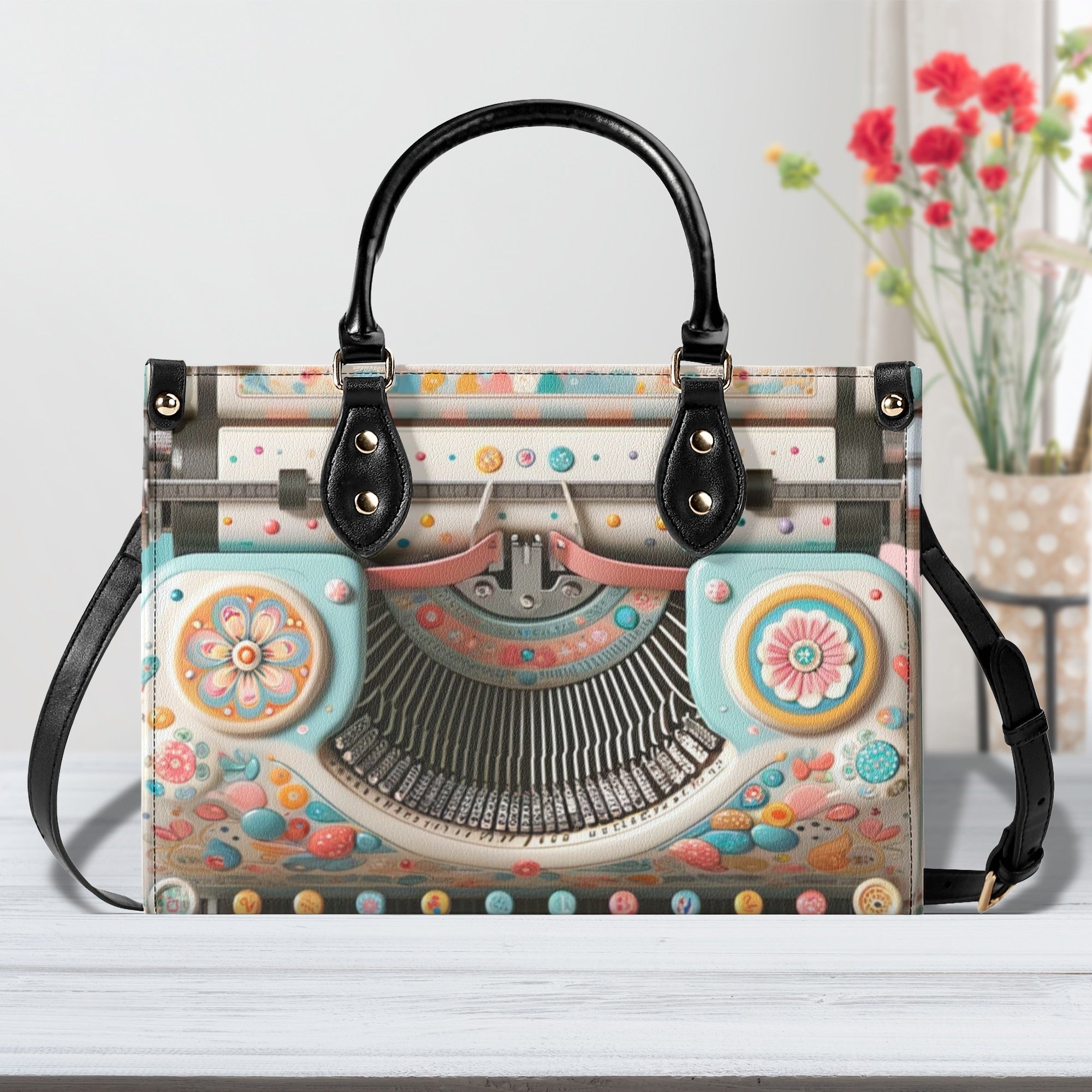The photograph showcases a unique purse designed to resemble a typewriter, with details that blend creativity and fashion. The purse is rectangular and features black leather handles centered at its top, as well as a black shoulder strap attached at the top left and right corners. The body of the purse is adorned with a typewriter key print, where each key is detailed with what it would print on paper. A vibrant mix of pastels and floral patterns, including shades of light blue, pink, and yellow, adorn the purse along with colorful dots and designs. It has two prominent circles with floral designs and metallic fixtures secured by pink clasps on the front. The backdrop of the image includes a pink vase with white polka dots, filled with red and yellow flowers, suggesting a home setting. The purse rests on a weathered wooden table, providing a rustic contrast to its eclectic and artistic design.